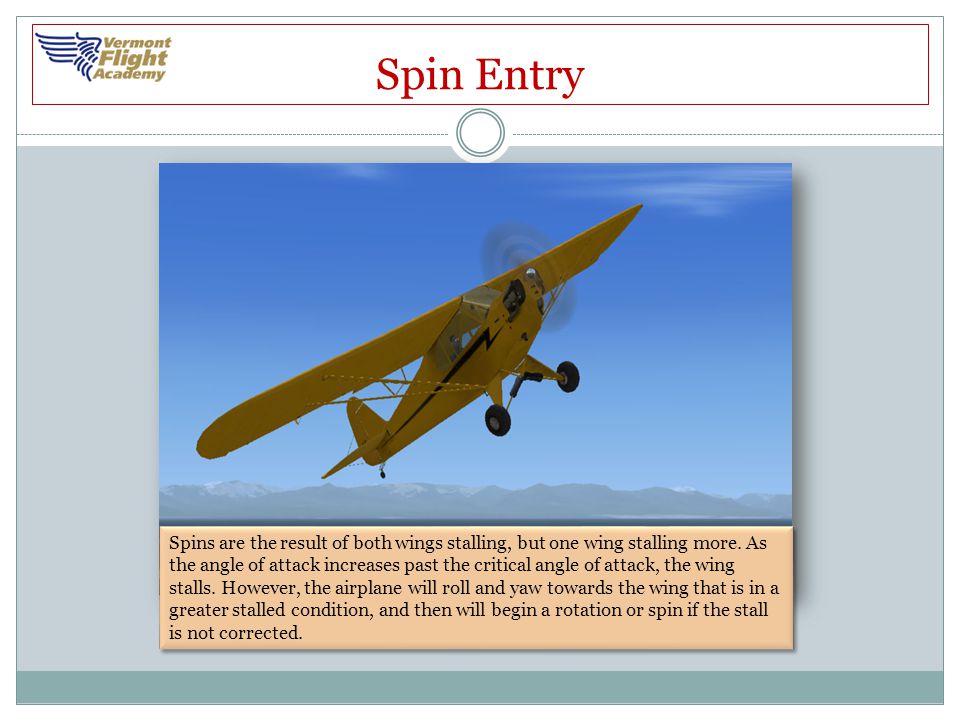The image is a detailed educational slide related to flying, featuring a small yellow Cessna aircraft with an overwing, single-engine, and a propeller at the front, angled upwards as if it is taking off. The backdrop offers a vivid blue sky with a mountain range visible at the lower level, providing a picturesque scene. The plane, detailed with a black stripe down its center and a distinctive 'Z' near the cockpit, is depicted starting a rightward roll which could lead to a spin if the stall isn’t corrected.

In the upper left corner, a logo with a blue wing and gold text reads "Vermont Flight Academy." The slide title, "Spin Entries," is displayed prominently in red at the top center. At the bottom is a detailed explanation on spins: “Spins are the result of both wings stalling, but one wing stalling more. As the angle of attack increases past the critical angle, the wing stalls. The airplane will then roll and yaw towards the wing in greater stalled condition, potentially beginning a rotation or spin if the stall is uncorrected.” The slide's overall aesthetic is enhanced by colors like white, red, blue, gold, and shades of brown, underlining its purpose as an educational tool.